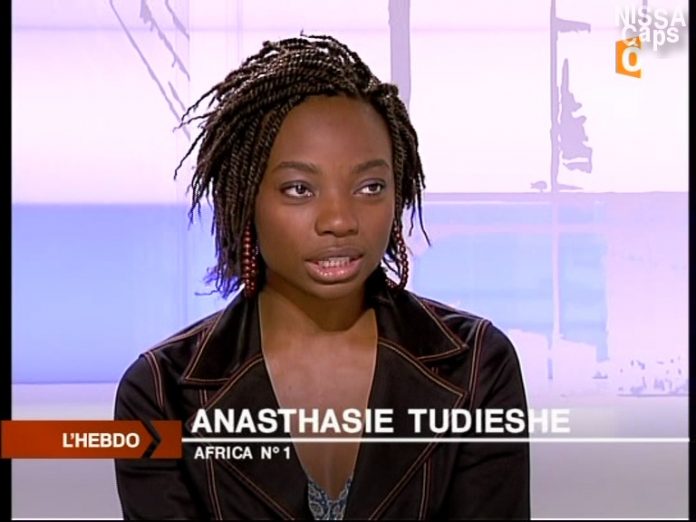In this image, the background features a stylized lilac mauve color with faint patches of baby blue, accentuated by lines and splotches of purple, creating a textured, square-like pattern. The top right corner of the image has a watermark that reads "Nyssa Caps" alongside a small orange logo with an "O". The main subject of the image is a black woman with dreadlocked cornrows, wearing a dark brown jacket over a low-cut blouse. The blouse is patterned in blue, white, and brown hues, peeking out at the V of her neckline. In the bottom left corner, a brownish-orange logo displays "Le Hebdo" with "Anastasie Tedeschi, Africa No. 1" written in white letters beneath it.